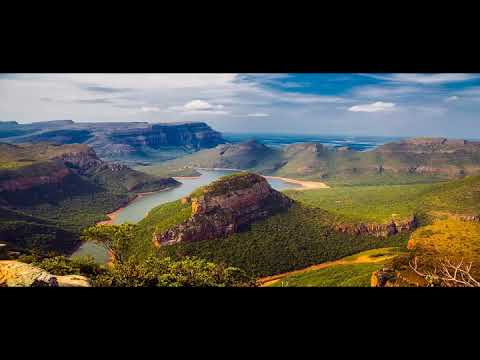An expansive scenic photograph captures a stunning landscape featuring a diverse topography of mountains, valleys, and waterways. In the foreground and center, a prominent butte rises, its base covered in lush green vegetation ascending to a rocky, light brown summit. The butte stands as a focal point amidst a sprawling valley where a river or lake of gray-blue water meanders gracefully. To the left, a ridge of green and brown mountains stretches from the left edge toward the center, terminating in an abrupt cliff that dramatically drops off. Beyond this ridge, a breathtaking view of an expansive ocean with dark blue waves dotted with white foam beckons in the distance.

The distant mountains gradually transform from vibrant greens to a bluish hue as they recede into the horizon. Overhead, a mostly cloudy sky casts a serene ambiance over the scene, with white clouds dominating the left side, while patches of gray intermingle with glimpses of pale blue sky on the right. Notably, in the bottom right corner of the image, some dead branches and vegetation contrast with the overall lushness, adding texture and depth to the composition. This photograph, taken during the daytime, masterfully captures the natural beauty and varied landscape of the region, showcasing both tranquil waterways and rugged highlands against the backdrop of a distant ocean and a cloudy sky.